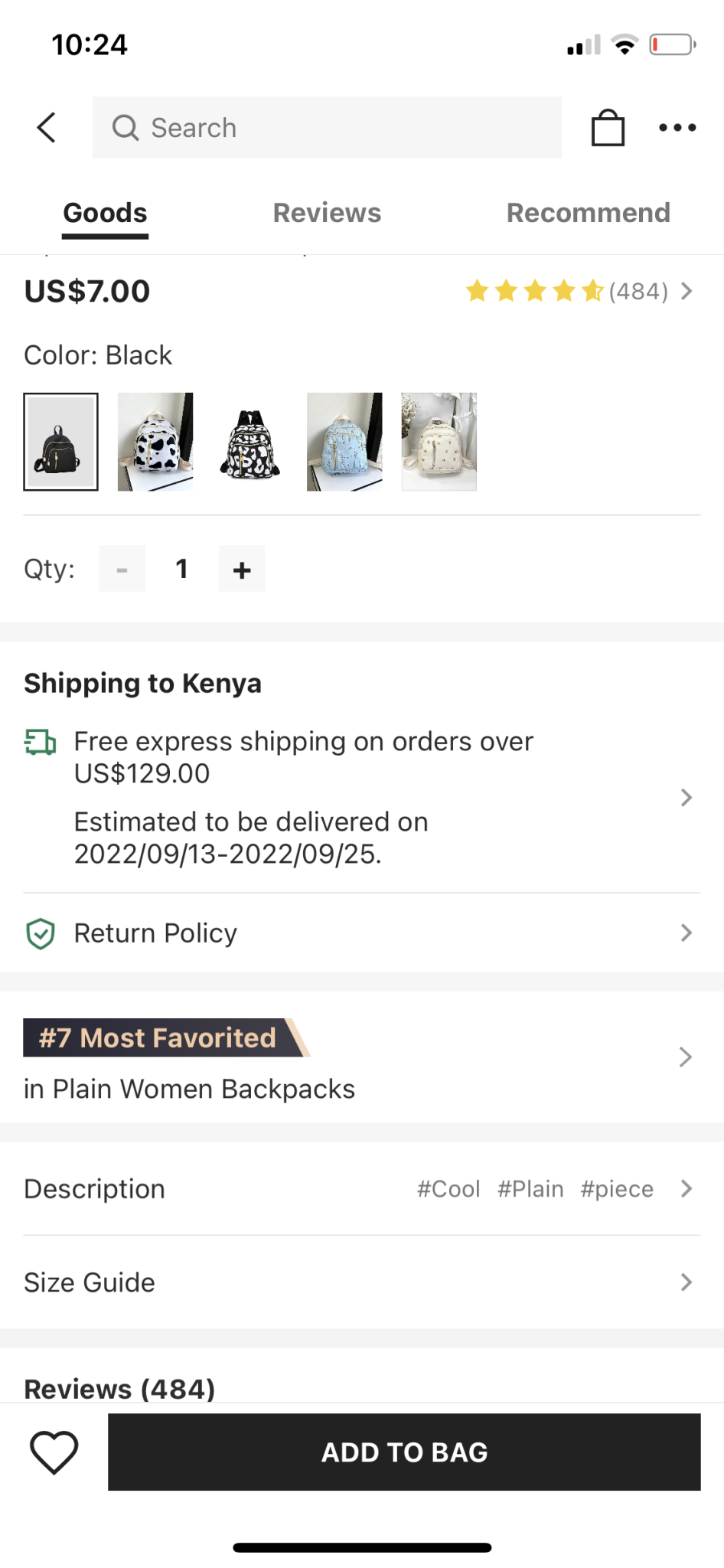The image depicts a detailed product listing for a black bag, presumably on a user's device. At the top of the screen, the status bar shows a battery icon in red, a left arrow, a gray Wi-Fi symbol with two signal bars missing, followed by a search icon. Below this, there are various product details including a gray underline.

The product listed is a black bag, featured multiple times within the image. Beside it, clear indicators for quantity adjustments show a plus sign to increase the quantity, and the current quantity set to one. Additionally, it specifies shipping details, stating that shipping to Kenya is available via Freight Express for $1.29, with an estimated delivery window between September 13, 2022, and September 25, 2022.

The listing highlights customer reviews with a rating of 4 stars out of 5, based on 484 reviews. It also mentions a price of $7.00. Further, the listing emphasizes the product as the 7th most favored in the "in-plane women backpacks" category and includes a brief description: "#cool, #plain, #peace".

Additional options include a size guide, the capability to view more reviews, and an option to 'add to bag' marked by a gray button with a hollow heart symbol indicating a wish list or favorite feature.